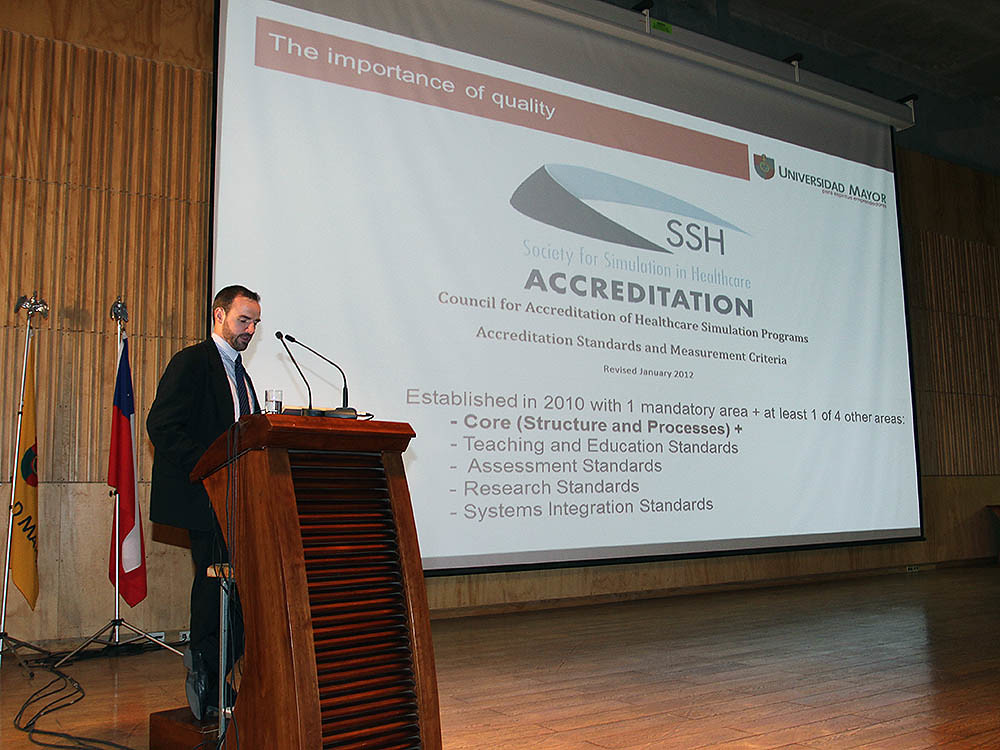A man in his early 40s, wearing a black suit, white shirt, and black tie, stands behind a dark wooden podium with two microphones on a hardwood stage. He has a beard and is speaking at what appears to be a convention. There are two flags behind him, one red and white and the other golden yellow with a black and red semicircle, both draped towards the ground on tripod poles. Behind the man, a large screen displays a detailed projection: at the top right, it reads "Universidad Mayor." Below that, a brown banner bears the text "quality" in white letters. The screen also displays the "SSH Society for Simulation in Healthcare" logo and the following text: "Council for Accreditation of Healthcare Simulation Programs, Accreditation Standards and Measurement Criteria, revised January 2012, established in 2010 with one mandatory area plus at least one of four other areas - core (structure and processes), teaching and education standards, assessment standards, research standards, systems integration standards." Behind the screen is a white, bamboo chute wall.